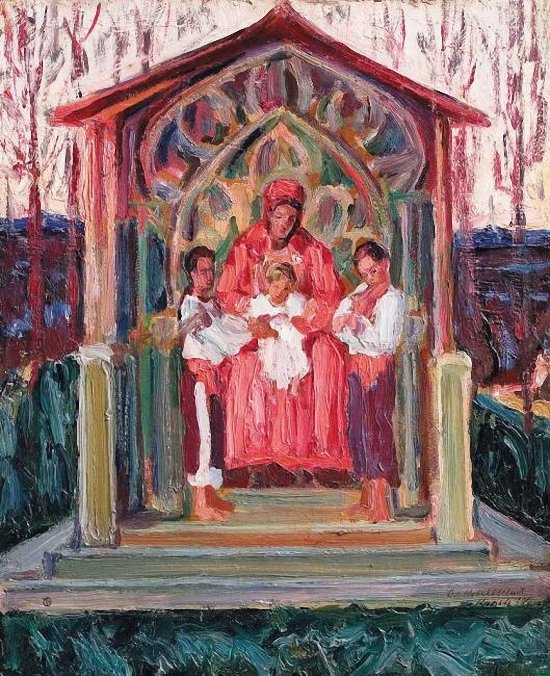In an impressionist, water-colored painting, a family is gathered together on a porch or pavilion that exudes a church-like aura. At the center, a mother dressed in a striking red dress and hat sits with one child, who is nestled on her lap and dressed in a white gown, with blonde hair and fair skin. To her left, a young boy stands, wearing a white shirt and unique pants that are black in the front with a white stripe down the side, transitioning to red in the back, and he is barefoot. On her right, a young man, also barefoot, plays a violin while dressed in a white shirt and pants that graduate from pink to blue and purple. The scene is outdoors, framed by a pointed red roof supported by yellowish-green columns, sitting on a gray and green concrete foundation surrounded by grass. Leafless trees with purple limbs stretch out in the background under a white sky, adding to the ethereal and somewhat abstract feel of the painting. The overall composition melds colors and forms in a way that suggests both realism and impressionism, creating a serene and nostalgic family tableau.